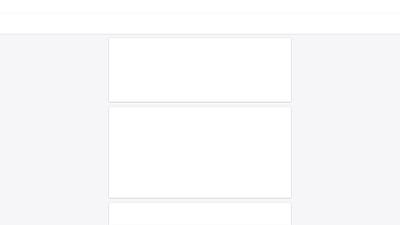The image appears to be a placeholder for a potentially unfinished or malfunctioning website. At the very top of the image, there is a pure white area, suggesting the presence of a title bar typically used to display the website name or title. This title bar would likely contain labels indicating the purpose of the page, positioned either to the left or center. On the far right side of this bar, there would be standard window control buttons for minimizing, maximizing, or closing the page.

In the central part of the image, there are three prominent rectangular areas, aligned vertically. These rectangles are potential sections where different types of information might be displayed. The rectangle in the middle is the largest, while the top and bottom rectangles are smaller, at approximately half the size of the middle one. Notably, the bottom rectangle is partially cut off, with only the first one-third visible within the image. Additionally, there are two gray areas located on the left and right sides of the central section, suggesting sidebars or additional segments that might be meant for navigation or supplementary content.

This placeholder image likely represents various sections of a webpage layout, awaiting further development or content.